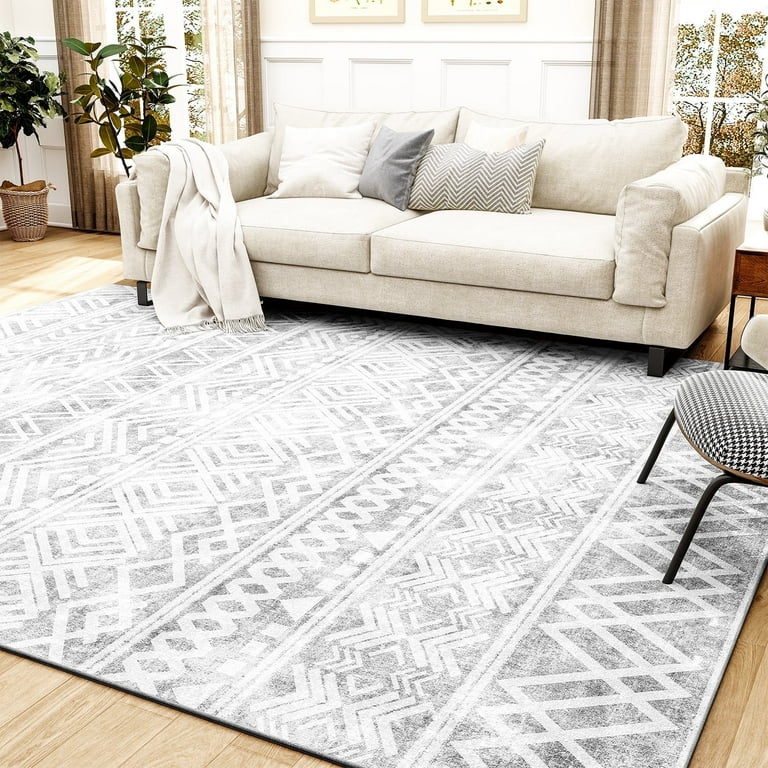This detailed, up-close interior photograph features a modern living room. Central to the image is a white couch, positioned horizontally against a white wall near the top of the photo. The couch is adorned with three cushions: a rectangular cushion with black zigzag patterns, a small rectangular gray pillow, and a plain white rectangular pillow. Draped over the left armrest of the couch is a white throw blanket. Behind the couch, two windows reveal a view of trees outside, and two potted ferns sit to the upper left in the frame. The floor is light-colored hardwood, partially covered by a large, gray and white area rug with geometric diamond and crosshatched patterns. A black and white checkered chair is partially visible on the far right, along with half of a mahogany end table. The scene is completed with an array of patterns on the couch, rug, and chair, creating a stylish and cohesive modern living space.